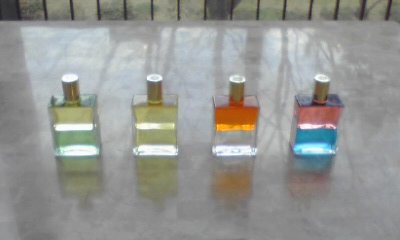The image features four bottles of perfume, each distinguished by its distinct color scheme and unified by their simple, square-shaped design with chrome lids. The bottles, absent of any labels or identifiable branding, are positioned side by side on a shiny, gray marble table that has black streaks running through it. The color combinations of the bottles, from left to right, are as follows: the first bottle is divided into pink on top and blue on the bottom, the second features orange on top and clear on the bottom, the third is uniformly yellowish-green throughout, and the fourth has yellow on top and green at the bottom.

The setting appears to be outdoors, suggested by the reflection of trees on the polished marble surface and the presence of a railing or fence visible in the background. This railing has slots through which green grass can be seen, and sunlight filters gently through the scene, creating subtle reflections and contributing to the overall serene atmosphere.